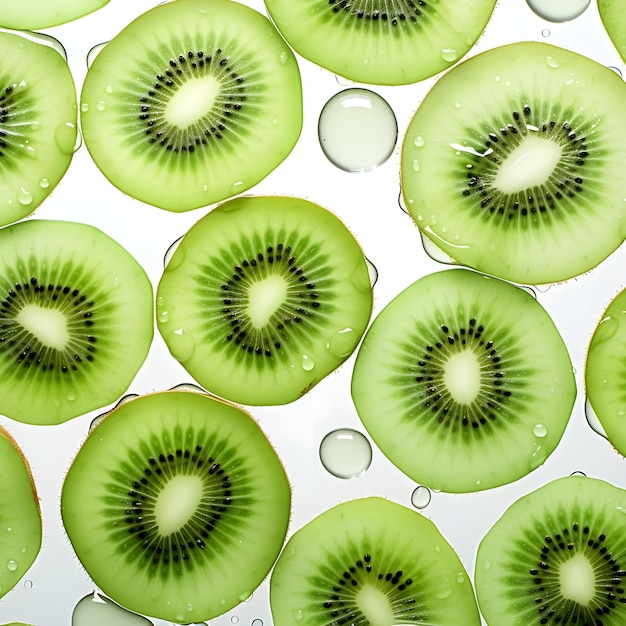The photograph features an arrangement of at least 15 thinly sliced kiwi sections spread evenly across a white, glass-like background. Each kiwi slice is a vivid light green, darkening towards the center where tiny, black seeds form a concentric pattern around an almost white core. The slices display a natural radial design, reminiscent of sun rays emanating from their centers. Some slices are fully peeled, revealing their smooth, green flesh, while others retain a portion of their brown, fuzzy skin, adding texture to the image. Scattered among the kiwi slices are large water droplets, with smaller droplets also clinging to some of the fruit surfaces, creating a fresh, dewy appearance. The water droplets and the white background, slightly tinted green by the kiwis, enhance the overall vibrant and refreshing aesthetic of the composition.